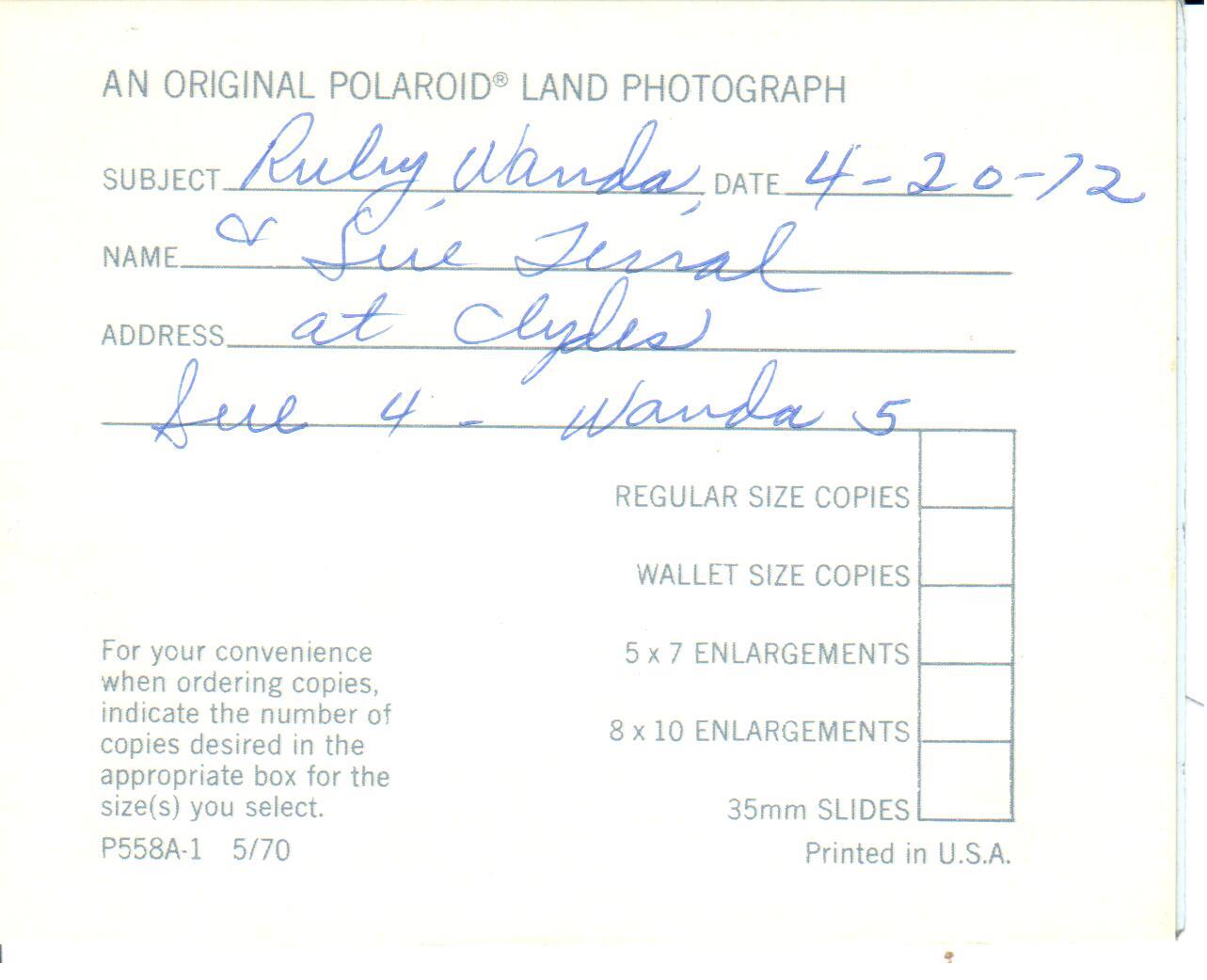The photograph depicts an old order form or record-keeping sheet for photographs, featuring a white background with black print at the top stating "An Original Polaroid Land Photograph." Below, the form is filled in with handwritten details in blue ink. The first line says "Subject," followed by "Ruby, Wanda" in cursive. The next lines show "Date: 4-20-72," "Name: Sue Terrell," and "Address: at Clyde’s." An additional notation reads "Sue for Wanda 5." Below the handwritten section, a blue typewritten paragraph instructs: "For your convenience, when ordering copies, indicate the number of copies desired in the appropriate box for the size you select. P558A-1, 5/70." Adjacent to this paragraph, the form features five empty boxes with corresponding lines labeled for different photo sizes: "Regular Size Copies," "Wallet Size Copies," "5x7 Enlargements," "8x10 Enlargements," and "35mm Slides." The form concludes with "Printed in USA" at the bottom.